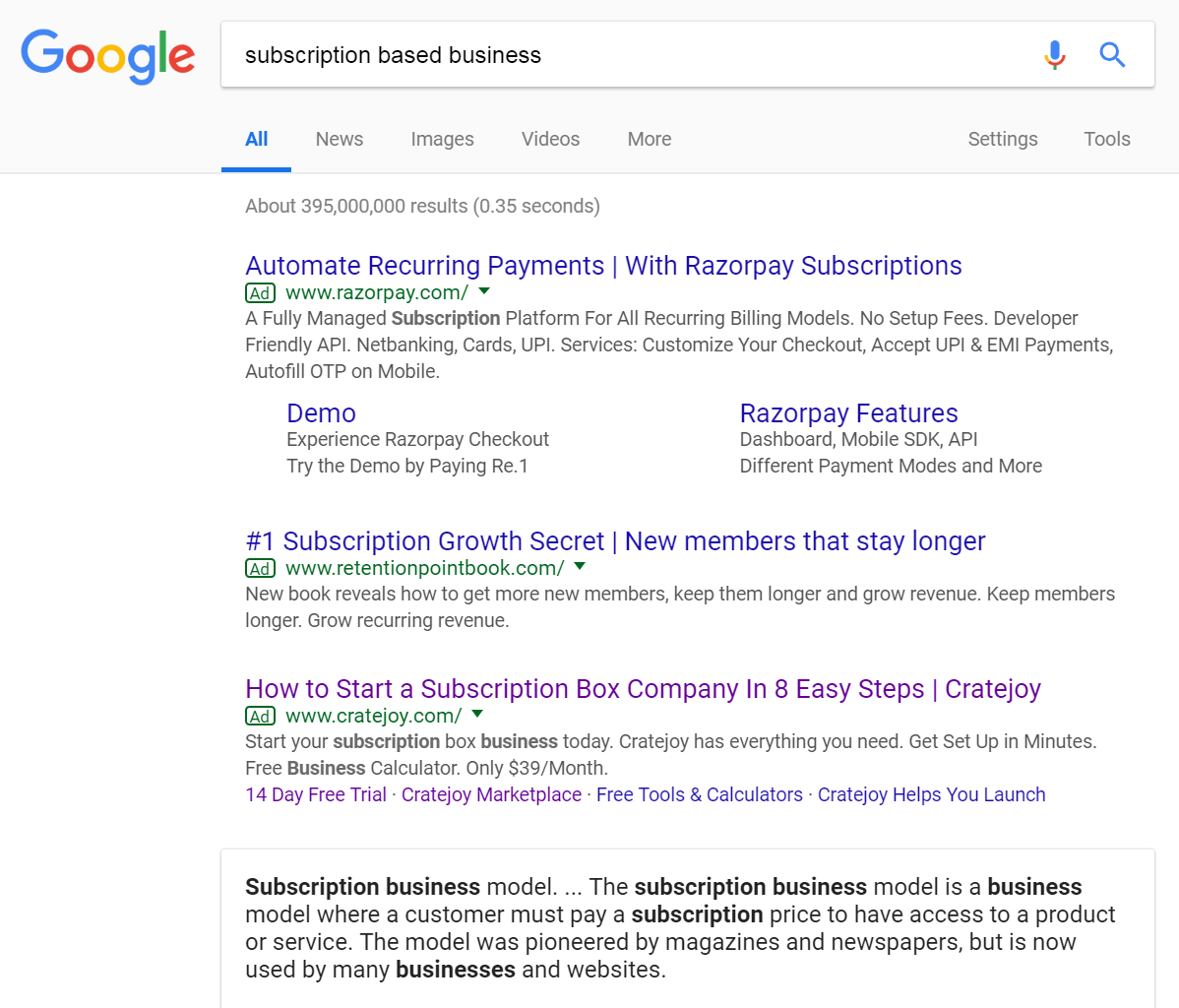The image displays a Google search results page. At the top, the Google logo is prominently featured in its iconic colors: blue, red, yellow, and green, within a gray rectangular background. Below this, inside the search bar, the phrase "subscription based business" is clearly visible.

Directly underneath, there is a navigational bar with the options "All", "News", "Images", "Videos", "More", "Settings", and "Tools". The "All" option is underlined and highlighted in blue, while the remaining options are in black, stretching horizontally from left to right.

The search results indicate approximately 395 million results. The first result is an advertisement with the headline, "Automate recurring payment with Razorpay subscriptions," followed by a brief black-text paragraph describing the service. Link prompts labeled "Demo," "Experience Razorpay checkout," "Try the demo by paying ₹1," and "Razorpay features" appear in blue.

Subsequent search results include:

- A link titled, "Number one subscription growth secret: New members that stay longer," in blue.
- Another link, "How to start a subscription box company in eight easy steps," from CreateJoy, also in blue.

A descriptive paragraph follows, explaining the subscription business model in black text: "The subscription business model is a business model where customers may pay a subscription price to have access to a product or service. The model was pioneered by magazines and newspapers but is now used by many businesses and websites."